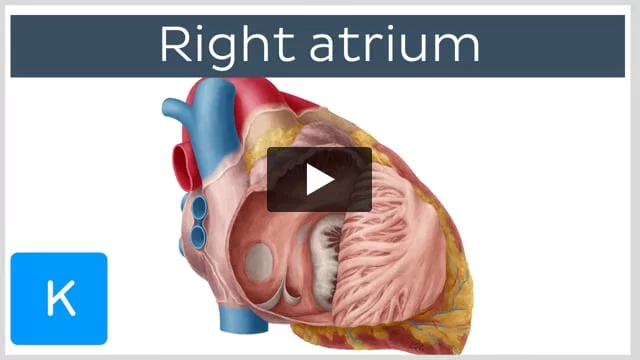The image is a detailed diagram of a human heart, depicting it in vivid colors and intricate detail. At the top of the image, there’s a band with "right atrium" written in white letters against a dark blue background. Central to the image is a dissected drawing of the heart, with various sections color-coded to highlight different parts. The heart itself is mostly flesh-colored, with a goldish hue and red at the top, representing different anatomical features like veins and tissues. Blue and red sections clearly distinguish the arteries and ventricles, enhancing their visibility. Additional highlights include a pink and yellow coloration, possibly representing muscle and fat layers. The diagrammatic heart is meticulously detailed to show internal structures, including white sections symbolizing veins and tissues. Positioned in the center of the image is a black box with a white play triangle, indicating it's a screenshot from a video. On the lower left-hand corner, there's a blue square with a white letter "K", set against a predominantly white background.